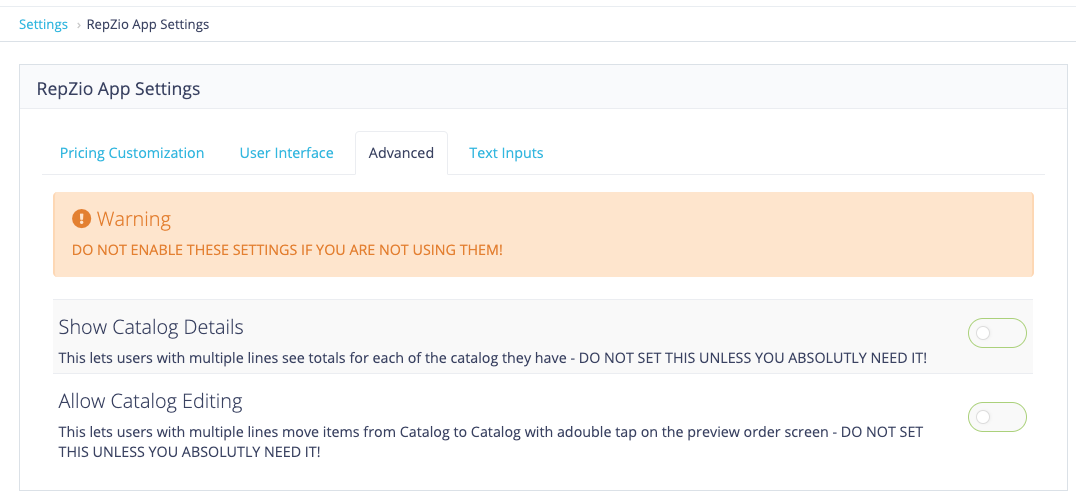In the upper left corner, the screen displays the word "Settings" in blue text, followed by "RepZio App Settings" in the same colored font. Below that, "RepZio" is repeated in black text, confirming it is indeed the settings for the RepZio app. Continuing down, the phrase "Pricing Customization" appears in blue text. To the right, the headings "User Interface" and "Advanced" are displayed in black text, with "Text Inputs" highlighted in blue text beneath them. 

A prominent long orange box on the screen features a dark orange circle with a white exclamation point inside, accompanied by a warning message in orange text: "Do not enable these settings if you are not using them!"

Further down, within a gray box, the option "Show Catalog Details" is listed, explaining that this feature allows users with multiple lines to view totals for each catalog they manage. This is followed by a bold caution: "Do not set this unless you absolutely need it." Lastly, the option "Allow Catalog Editing" is detailed, indicating that it enables users to move items between catalogs with a double tap on the preview order screen. This comes with a similar bold warning: "Do not set this unless you absolutely need it!" and is punctuated with an exclamation point for emphasis.